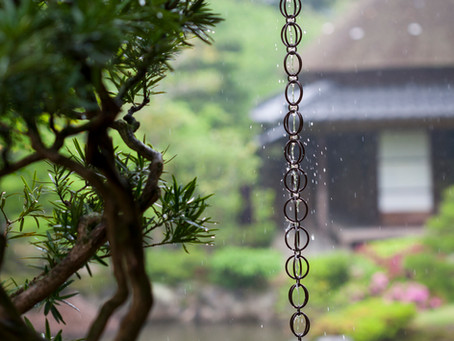In the foreground of this photograph, a close-up of a finely detailed spiky green bonsai bush or tree branch dominates the left side, showing off its meticulously trimmed brown branches and vibrantly sharp needles. Nearly centered, but leaning towards the right side of the image, a chain made of round brass links, each interconnected with smaller circular links, captures the eye. This chain, possibly part of a wind chime or bird feeder, appears to be in motion, with water droplets spraying and splashing off it, suggesting it’s raining or that water is running through it. The motion blur gives a dynamic sense of movement to the image. The background, rendered in a soft blur, features a brown house with a white window and metal roof, surrounded by green foliage, flowers, and bushes, which lend a lush, natural atmosphere to the scene. The combination of sharply focused foreground elements against the diffused background provides a striking contrast, creating a vivid and dynamic image.